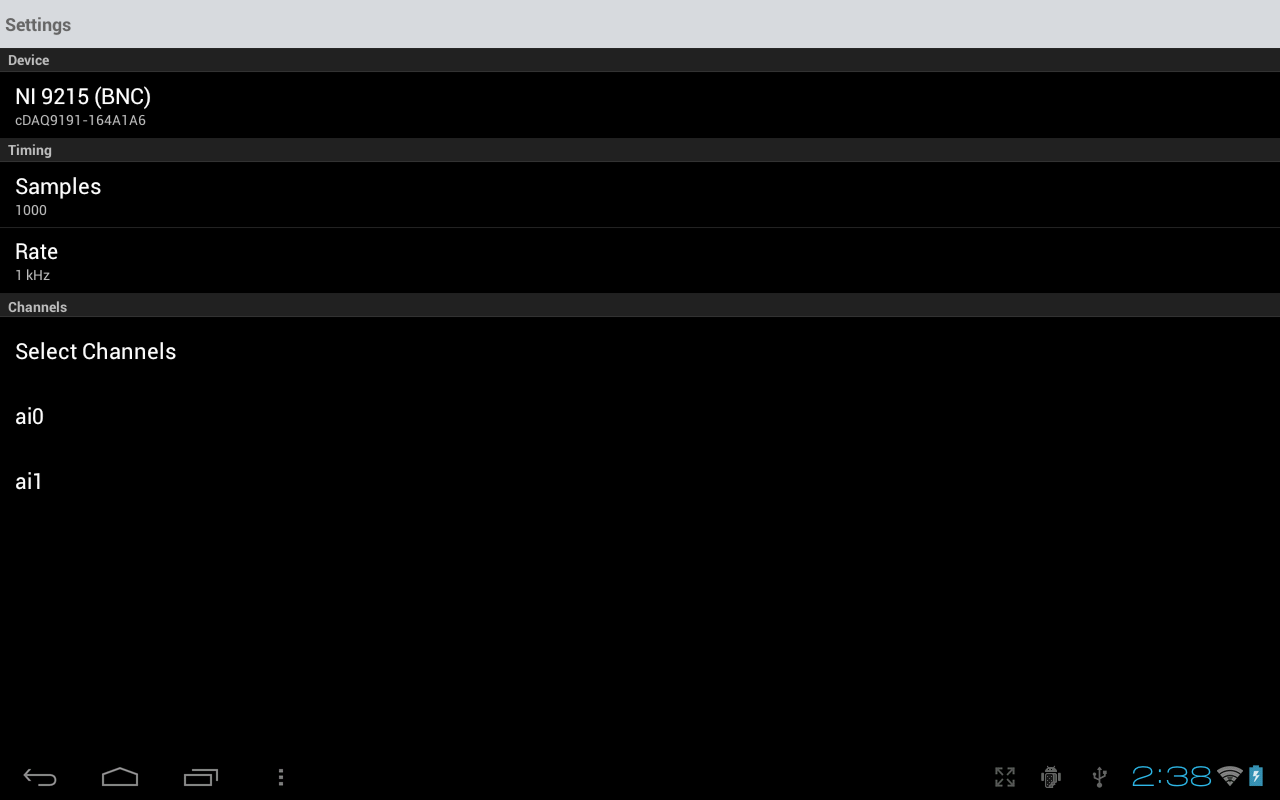Here is a detailed and cleaned-up version of the caption:

---

The image is a screen capture displaying the settings interface for a specific program or device. At the top, a gray bar prominently features the word "Settings." Below this, the main content is set against a black background, which occupies the majority of the screen. 

At the bottom of the black background, there is a navigation bar starting with a back arrow, followed by a stylized home button, and a button representing multiple screens. Further to the right, there is a menu icon, and then an icon designated for screen expansion or additional functions, which is not clearly visible in this capture. 

On the far right of this bottom bar, several indicators are displayed: a USB symbol, the current time (2:38), signal strength, and a battery strength indicator.

The settings interface lists several sections:
1. **Device**: This specifies the device name and type, which in this case is "BNC."
2. **Timing**: Under this section, the number of samples and the sample rate are detailed.
3. **Channels**: Here, you can select different channels, which are divided into two options: AI0 and AI1.

This comprehensive view encapsulates the featured options and indicators on the settings screen for the program or device.